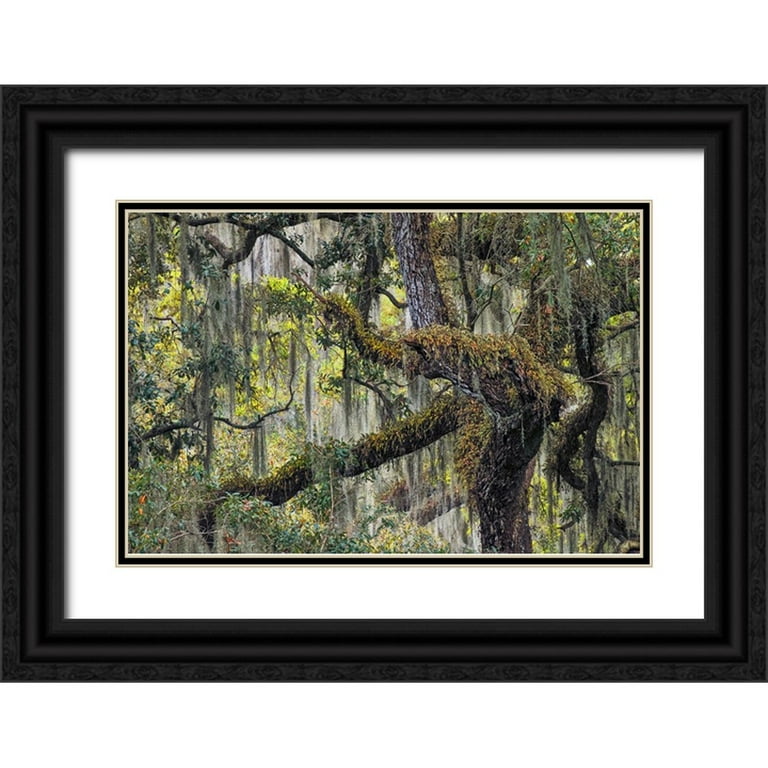The artwork is a mounted wall piece featuring a photograph or drawing of an outdoor scene, either a swamp or rainforest, displayed on a white wall. The image is enclosed in a rectangular, solid black frame that might be wooden, surrounded by a plain white border and a smaller black border. In the center, the focal point is a large tree with a dark brown trunk on the right side. Greenish-orange moss carpets the tops of the branches, adding a textural element, while green vines drape themselves over the branches from the top of the frame. The backdrop is bathed in daylight, evidenced by brighter, grey-green leaves. The overall composition highlights a tangle of branches and foliage, balancing darker and lighter shades of green that create a dynamic contrast within the dense forest setting.